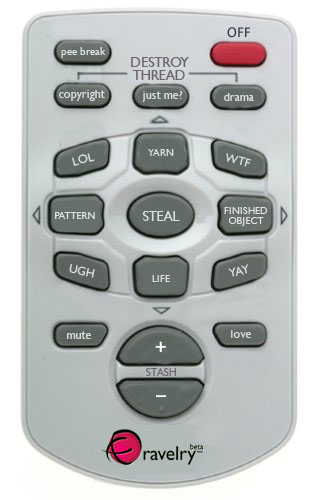The image depicts a light gray television remote control branded with "Ravelry Beta" at the bottom. The remote is relatively short and features a range of uniquely labeled buttons in dark gray, with a single red "off" button located in the upper right-hand corner. At the top center of the remote, the label "Destroy Thread" is noticeable. The buttons are arranged as follows:

- The top row contains two buttons: "P-Brake" on the left and the red "off" button on the right.
- Below this row, there are three gray buttons labeled "Copyright," "Just Me," and "Drama."
- In the middle section, nine buttons are arranged in a directional pad orientation with the labels: "LOL" at the top, followed by "Yarn," "WTF," "Pattern," "Steel," "Finished Object," "Ugg," "Life," and "Yay."
- Near the bottom, there are buttons for "Mute" on the left and "Love" on the right.
- At the very bottom, there are "plus" and "minus" buttons with the word "Stash" positioned centrally between them. 

This remote combines a quirky assortment of text, offering a playful twist on traditional remote control designs.